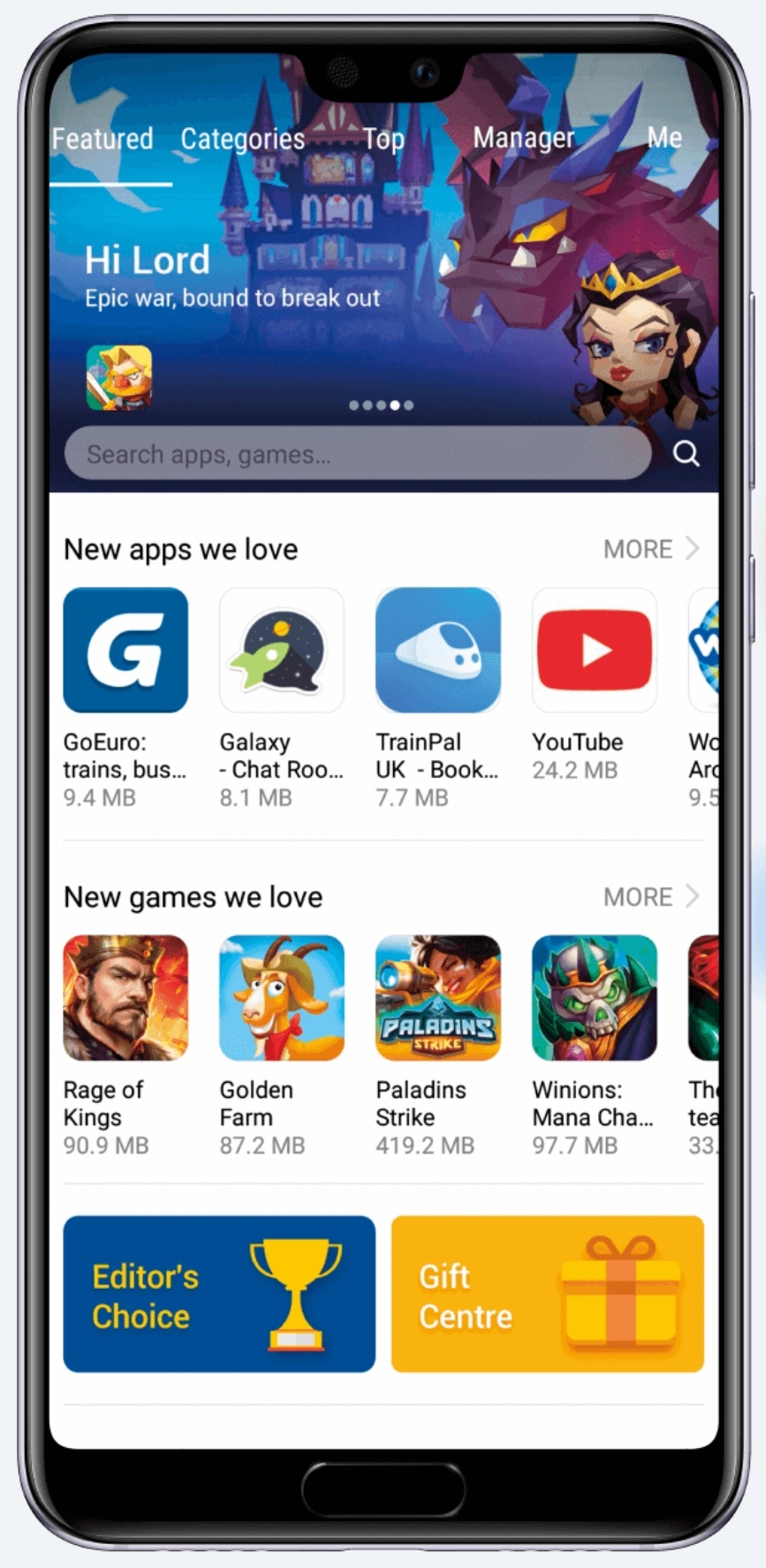A smartphone screen displays the Google Play Store interface. At the top are several tabs including "Featured," "Categories," "Top Manager," and "Me," with the current view set to the "Featured" section. Below the search bar, a prominent advertisement for a game titled "High Lord: Epic War" catches the eye. The ad features striking imagery, with a castle in the background, a woman in the foreground, and a playful dragon companion. Scrolling down, the section titled "New Apps We Love" showcases apps like "Go Euro," a metro-related application, "Galaxy Chatroom," "TrainPal," and "YouTube." Further down, the "New Games We Love" section includes titles such as "Rage of Kings," "Golden Farm," and "Paladin Strike." As you continue, there's an "Editor's Choice" or "GIF Centre" section, notable for its British spelling of "Centre." The overall design maintains a clean, white background, characteristic of a typical app store layout.